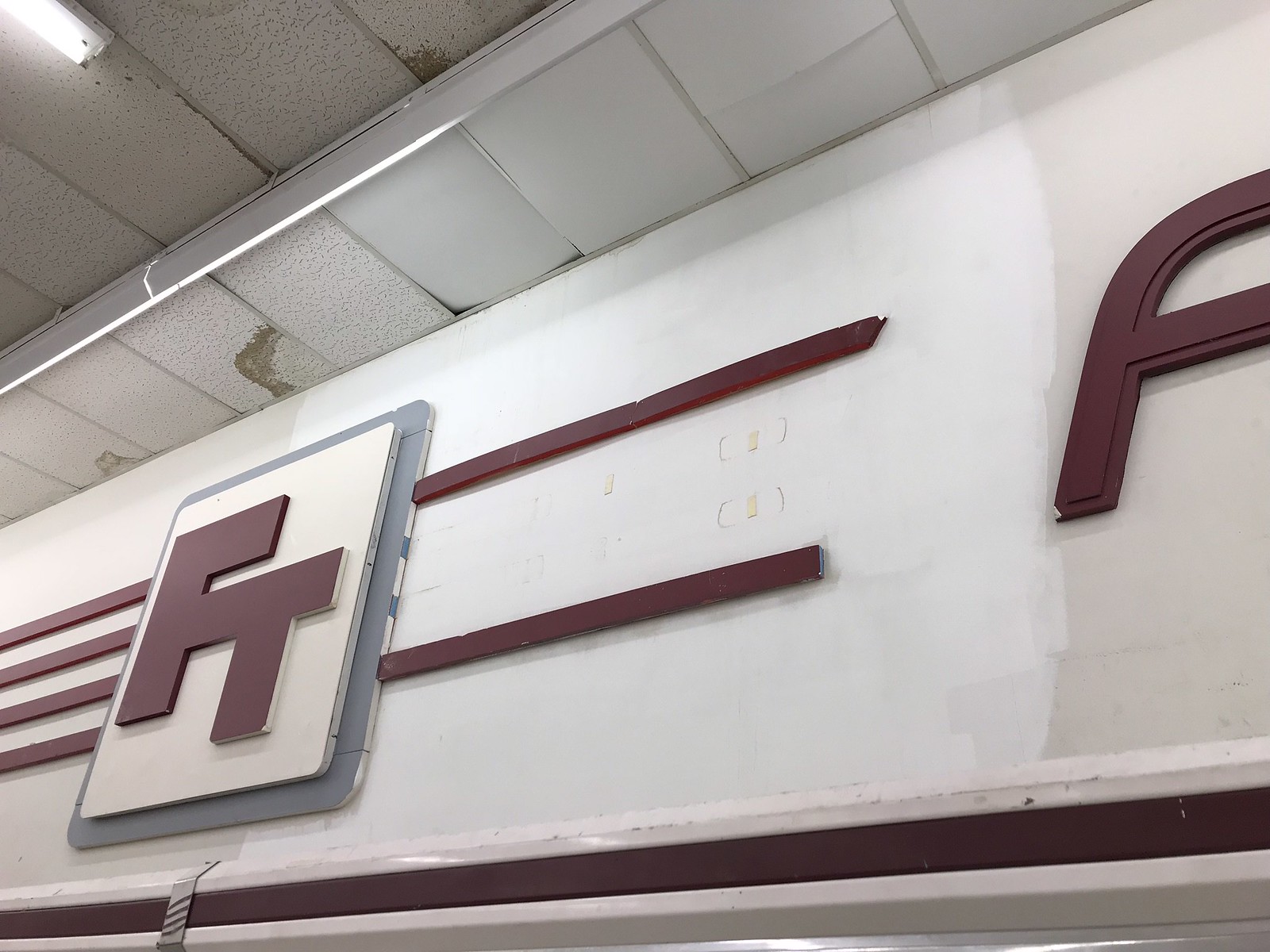The colour photograph captures an interior space, viewed looking upward towards the ceiling and the top of a wall. The ceiling features a drop-style structure with tiles in various states of wear: some are plain white, while others are a less brilliant white dotted with dark speckles. Many tiles show signs of age, including brownish stains and horizontal breaks. An illuminated strip light is partially visible in the top left corner.

On the back wall, a sign dominates the scene. The sign comprises a grey plate mounted on the wall, with a white rectangular plate layered on top. Central to this is a maroon symbol resembling a capital 'F' with a horizontal line intersected by a 'T,' suggesting it reads 'FT.' To the right edge of the sign, cut off by the frame, an element that might be the beginning of a capital 'A' or a lowercase 'f' is visible.

The overall environment appears commercial, though it's unclear if it's a store or perhaps a train or airport station. The wall with the sign looks like it could use cleaning, and the ceiling suggests the need for maintenance, likely from unresolved roof leaks. The setting gives a sense of a well-worn, utilitarian space.